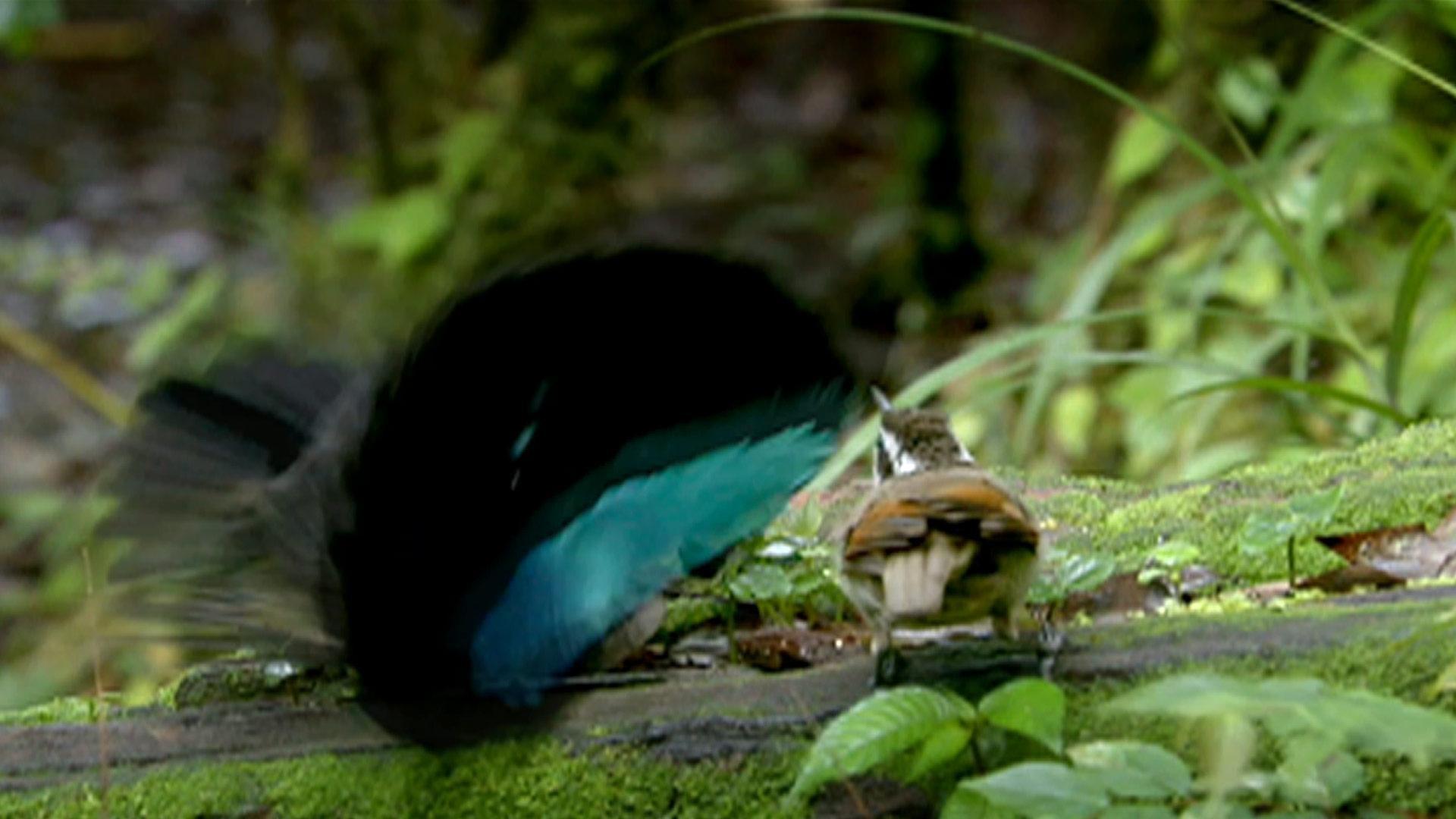In this detailed outdoor photograph, we see two birds positioned amidst a serene, shallow aquatic environment surrounded by lush, leafy green vegetation of varying shades. The foreground features a piece of stone with algae and foliage growing on it. One bird, likely a grouse, stands atop a fallen tree. This bird has a distinct appearance, with a brown tail, rust-colored wingtips, and predominantly brown plumage. Its head is adorned with brown feathers on the top, and white feathers along its neck sides. The grouse has black legs and feet and is observing another bird. The other bird, positioned slightly towards the left, appears blurred due to motion. Its plumage showcases a combination of teal blue, black, and gray feathers, with the tail feathers spread out prominently. The serene backdrop blurs into more dense vegetation, enhancing the focus on the avian subjects. Rocks and shallow water enhance the natural, tranquil setting where these birds interact.